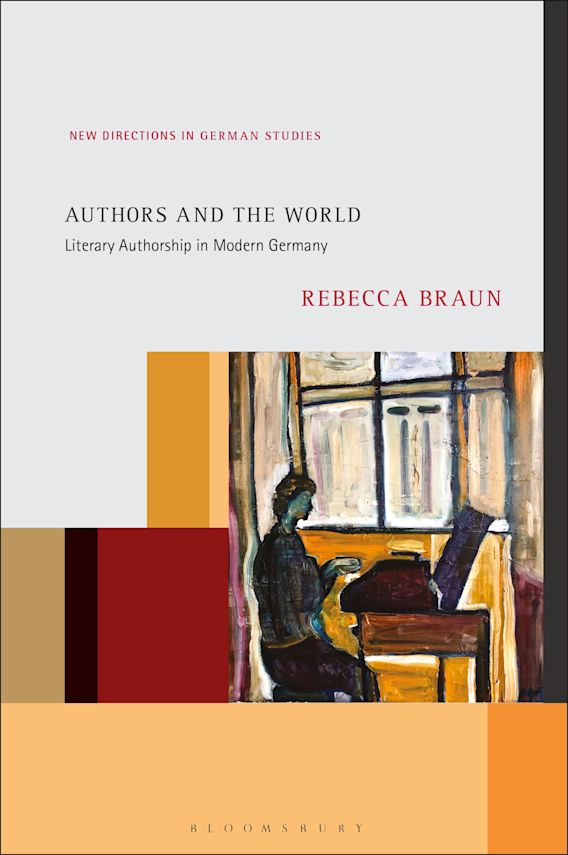Vertical rectangular book cover with an abstract design. At the top, against a gray background, the title "New Directions in German Studies" is written in red, slightly left of center. Below it, in larger black text, is "Authors and the World" followed by "Literary Authorship in Modern Germany" in slightly smaller black text. Further down to the right, in prominent red letters, is the author's name, "Rebecca Braun."

Beneath this text, there is an abstract painting depicting a person seated at a wooden desk with a typewriter, facing the right. The scene includes a window behind the person, suggesting light entering from outside. To the left of this image, the background features a blend of colors including yellow, orange, gray, red, dark brown, and tan, with these hues extending to the edges of the cover.

Towards the bottom in the middle, some additional text is discernible, potentially including the publisher's name, "Bloomsbury." The painting and the multicolored rectangles create a layered, artistic effect.